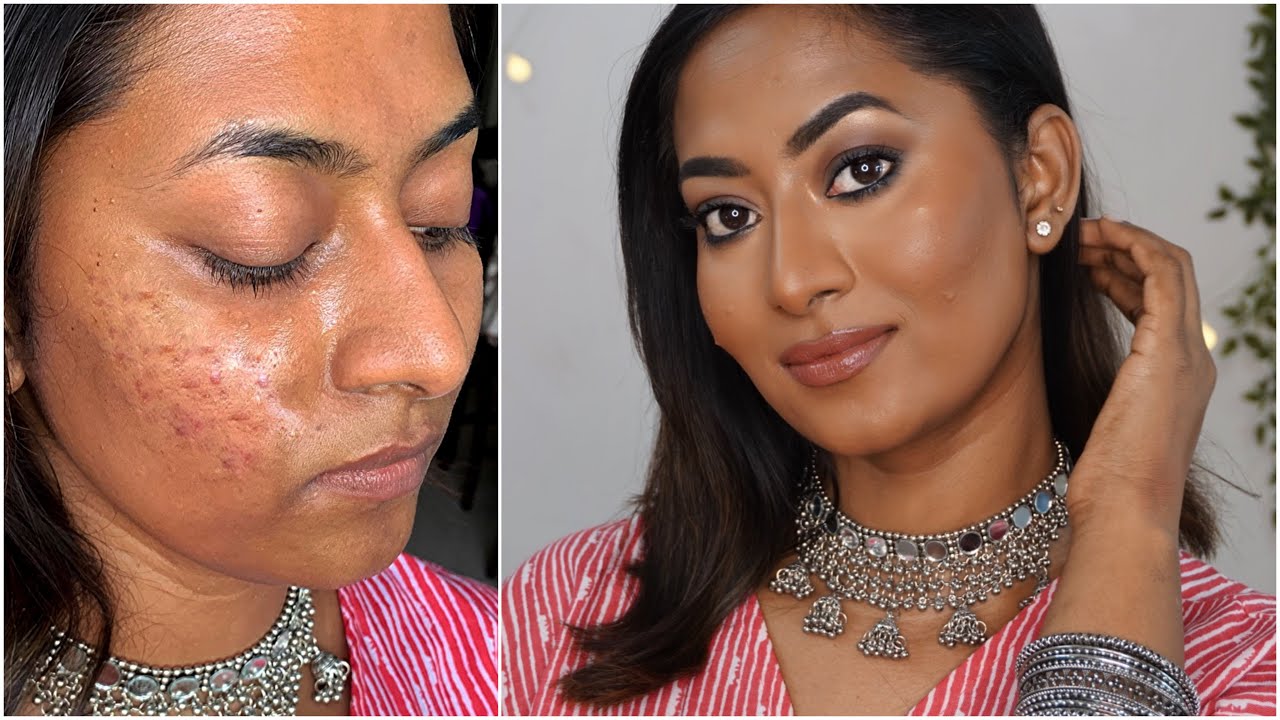This collage features a transformative beauty before-and-after set of a South Asian woman with a darker complexion and long black hair. The left image is a side-close-up of her with her eyes looking down, showcasing her natural state sans makeup, highlighting her noticeable acne and red marks on her cheeks. She adorns a silver necklace and a red and white V-neck outfit. Contrasting vastly, the right image captures her with a flawless face graced with comprehensive makeup, enhancing her eyes, eyebrows, and lips. Her complexion appears smooth and luminous, effectively concealing her acne. She faces forward with her brown eyes open, donning circular earrings with white stones and silver bangles. The background on the right is white, complemented by a potted plant, emphasizing the dramatic and significant transformation achieved through makeup.